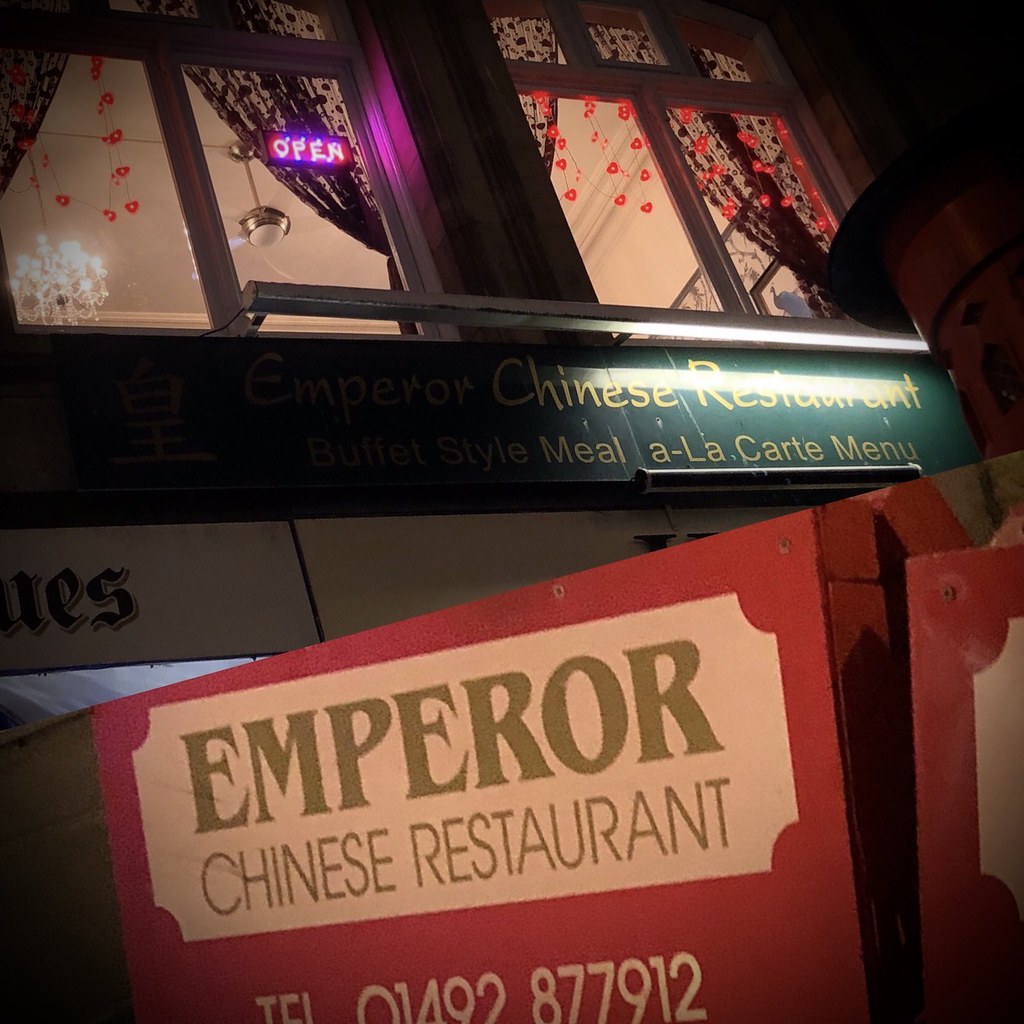This nighttime outdoor photograph captures the front facade of the Emperor Chinese Restaurant. The focal point is a vibrant red and white sign at the bottom of the image, designed in a ticket shape, with green letters that spell out "Emperor Chinese Restaurant." Below this, the telephone number "01492 877912" is prominently displayed. Above this sign, on the building’s facade, a larger dark green sign with gold text advertises "Chinese Restaurant, Meal, a la carte menu." Illuminated by a fluorescent bulb, this sign stands out in the night. The window above the signs features sheer lacy curtains, an eye-catching pink neon "open" sign, and red garland decorations that resemble hearts, adding a festive touch. In front of the restaurant, there is also a curbside wooden blackboard sign, typically used to display daily specials. The two combined photographs highlight the distinctive and welcoming appearance of this Chinese eatery.